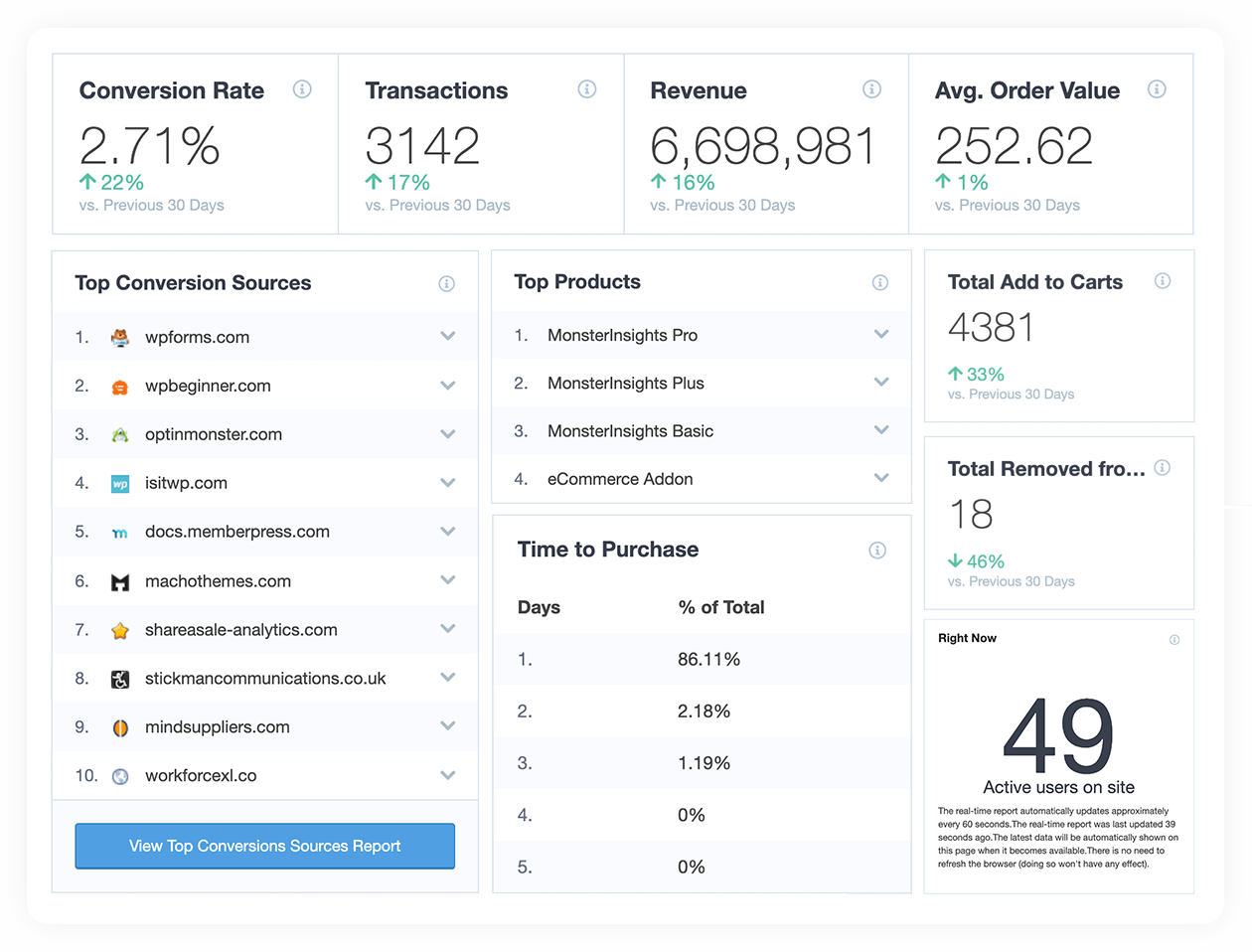**Screenshot Overview of Web Analytics Dashboard**

The image is a screenshot of a web analytics dashboard, characterized by a clean and organized interface with a faint gray outline enclosing a predominantly white background. The dashboard is compartmentalized with sections having bluish-gray shades.

**Top Metrics:**
- The top section extends almost the entire width of the screen, divided into four equal parts, each labeled with bold black text:
  - **Conversion Rate**: 2.71% (Up 22% from the previous 30 days), indicated by a blue information circle.
  - **Transactions**: 3,142 (Up 17% from the previous 30 days).
  - **Revenue**: $6,698,981 (Up 16% from the previous 30 days).
  - **Average Order Value**: $252.62 (Up 1% from the previous 30 days).

**Left Column:**
- Contains a dropdown box labeled in bold black text:
  - **Top Conversion Sources**: Listed from 1 to 10 with respective icons:
    1. wpforms.com
    2. wpbeginner.com
    3. optinmonster.com
    4. isitwp.com
    5. docs.memberpress.com
    6. macothemes.com
    7. sharesale-analytics.com
    8. stickmancommunications.com
    9. mysuppliers.com
    10. workforcexl.com

**Middle Column:**
- Comprises two stacked boxes:
  - **Top Products**: Bold black heading listing four products:
    - Morning Insights Pro
    - Morning Insights Plus
    - Morning Insights Basic
    - eCommerce Add-on
  - **Time to Purchase**: Bold black heading with days and their respective percentages:
    1. 86.11%
    2. 2.18%
    3. 1.19%
    4. 0%
    5. 0%

**Right Column:**
- Contains three boxes:
  - **Total Add to Cart**: Bold black heading with 4,381 (Up 33% from the previous 30 days).
  - **Total Removed From Cart**: Bold black heading with 18 (Down 46% from the previous 30 days).
  - **Active Users**: 49 current active users on the site, with additional details in smaller black text underneath.

**Visual Indicators:**
- Arrows indicating changes are green, signifying positive changes, with corresponding percentages also in green.

This detailed breakdown provides an insightful and comprehensive view of the web analytics dashboard's key metrics and data visualizations.